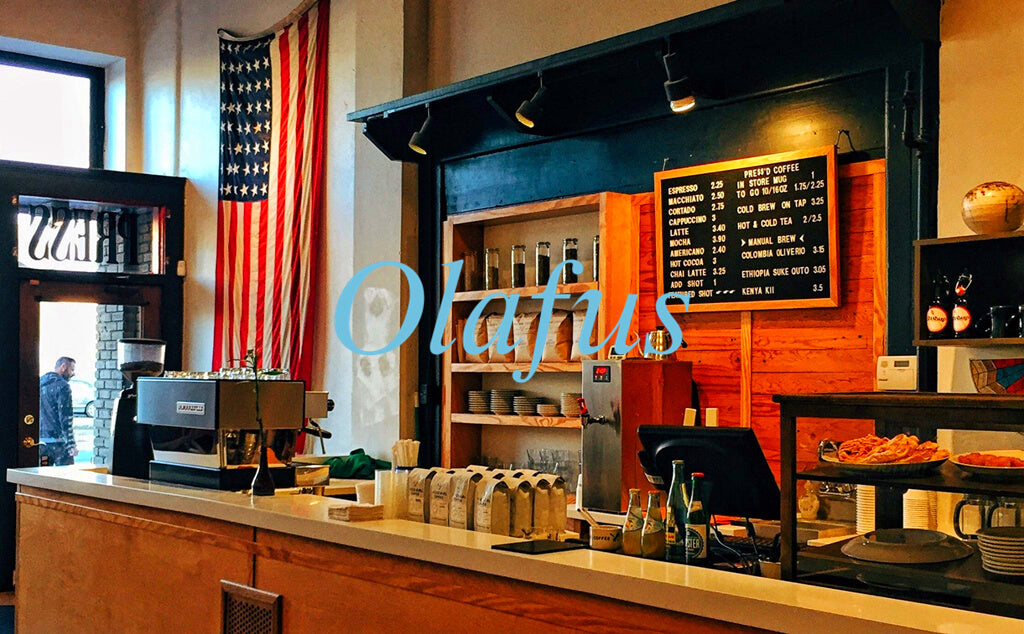The photograph captures the lively interior of a coffee shop named "Olafas" prominently displayed in baby blue text at the center. The scene is set against a white wall adorned with an American flag to the left, adding a patriotic touch. Below the flag, the glass entrance door is visible, with a passerby in a hoodie seen outside. The counter spans the entire width of the image's foreground, showcasing a variety of items including plates of food, cakes, and an array of drinks. Behind the counter, a detailed menu board lists various coffees, such as espressos priced at $2.25, macchiatos, Americanos, and teas. To the left of the counter, shelves stocked with glass containers, plates, and bags of coffee beans ready for grinding can be seen. The area is illuminated by three overhead lights, casting a warm glow on the assortment of goods displayed beneath, including a cash register and pre-made coffee bags. A cozy representation of a bustling coffee shop where customers can place their orders and enjoy a variety of beverages and treats.